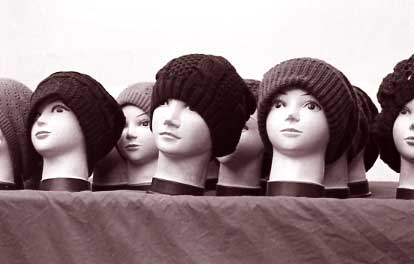The photograph depicts a collection of around eleven detailed female mannequin heads, each adorned with various knitted beanies, arranged on a surface draped with a mid-brown cloth that reveals creases. The image is visually distinct due to a brownish sepia filter, enhancing its vintage aesthetic akin to a black-and-white photo with brown undertones. The mannequin heads, all bearing delicately painted features including eyes, lips, and eyebrows, possess pale "skin," and are aligned in a slightly staggered manner, giving the impression they are facing somewhat towards the camera while slightly turned away. Each beanie varies in texture and style; some showcase ribbed circumferences of different depths, others exhibit shorter ribbing or additional patterns like crosshatching, and a few might feature small decorative elements such as flowers. Additionally, a thin ribbon is visible around the neck area of the mannequins, adding to the intricate display. The upper portion of the image is significantly overexposed, eliminating any contextual background detail and leaving the setting ambiguous.